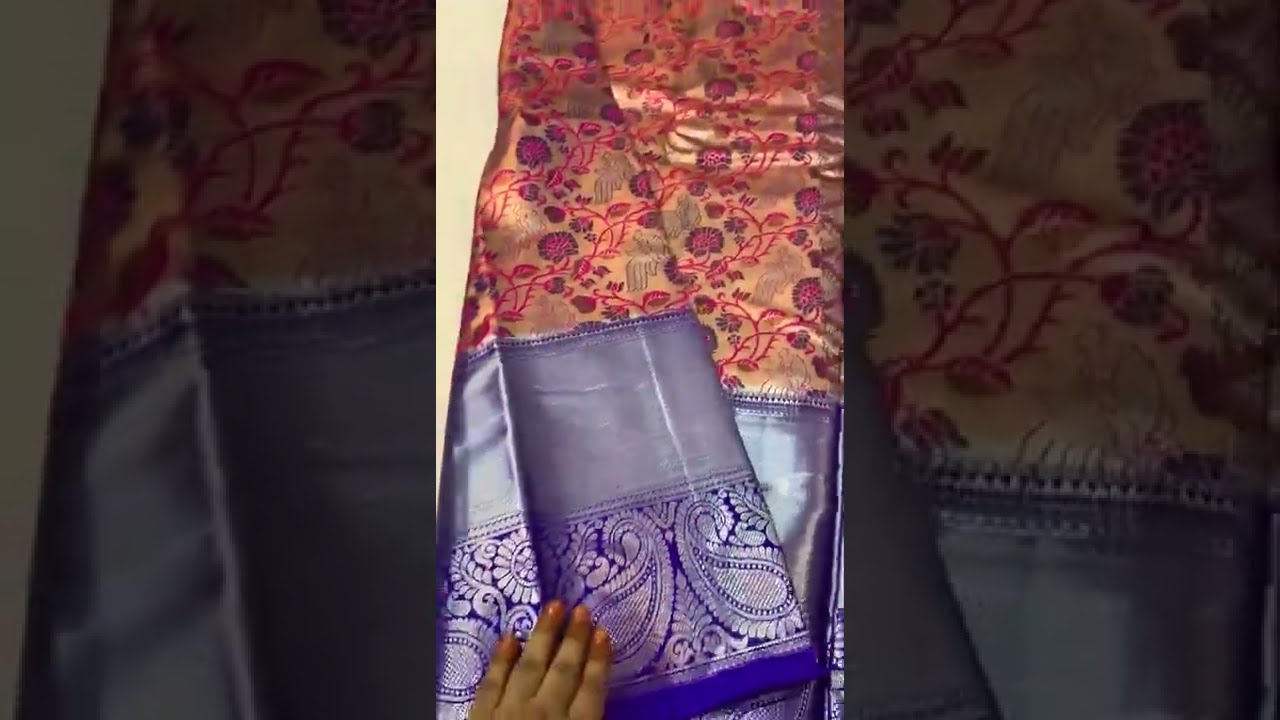This image is a vertical rectangular snapshot, likely a screen grab of a vertical video displayed on a computer screen with the central third clearly visible and the side thirds echoing the central image in a darkened, zoomed-in manner. The focus is a segment of a traditional Indian garment, possibly a sari or an elaborate robe. The upper section of the garment features a yellowish-peach background adorned with intricate red, green, and gold floral designs, including patterns resembling plants and puffed flowers with reddish hues and brownish accents.

A woman's hand with light peach nail polish enters from the bottom edge, interacting with the fabric. The bottom of the garment prominently displays a rich, dark blue band made of what appears to be a satin-like fabric. Below this, an elaborate paisley or filigree pattern is visible, executed in various shades of blue from dark and bright to soft tones. The design elements in the lower part also include henna-style motifs on a dark purple base, transitioning into slightly lighter purple sections, enriching the complexity and elegance of the fabric.